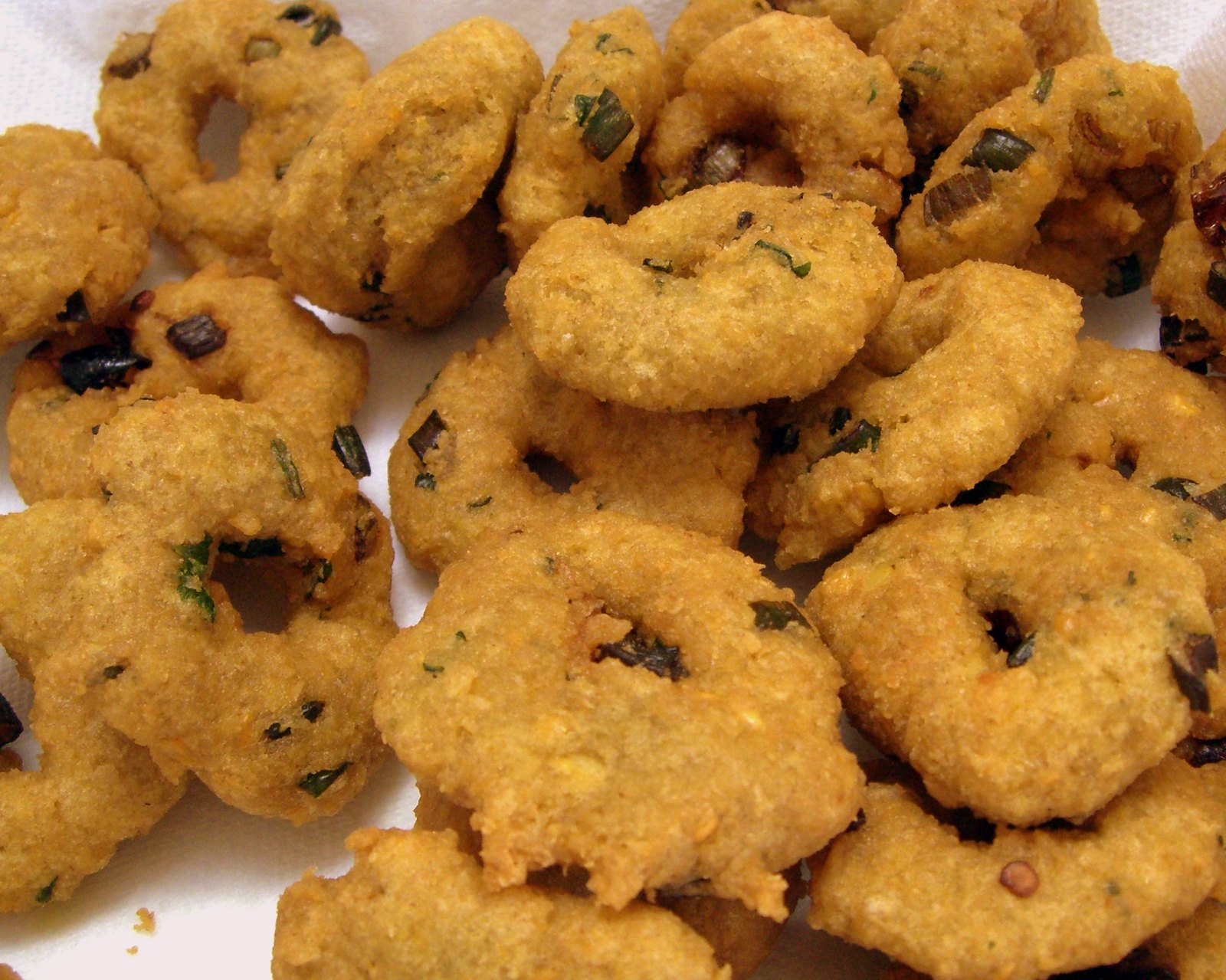This close-up photo displays a delectable pile of deep-fried onion rings, showcasing their crispy, golden-brown batter interspersed with hints of darker, slightly charred onion peeking through in spots. These rings are stacked on what appears to be a white paper towel, likely used to soak up excess oil after frying. The rings vary in appearance; some feature characteristic round holes, confirming their identity as onion rings, while others appear more filled in. Crumbs of the crispy batter, some of which seem to contain flecks of herbs and parsley, have fallen to the bottom left corner, adding texture to the presentation. In the foreground, three distinct onion rings are clearly visible, with more clumped together in the background, particularly towards the top right of the image.